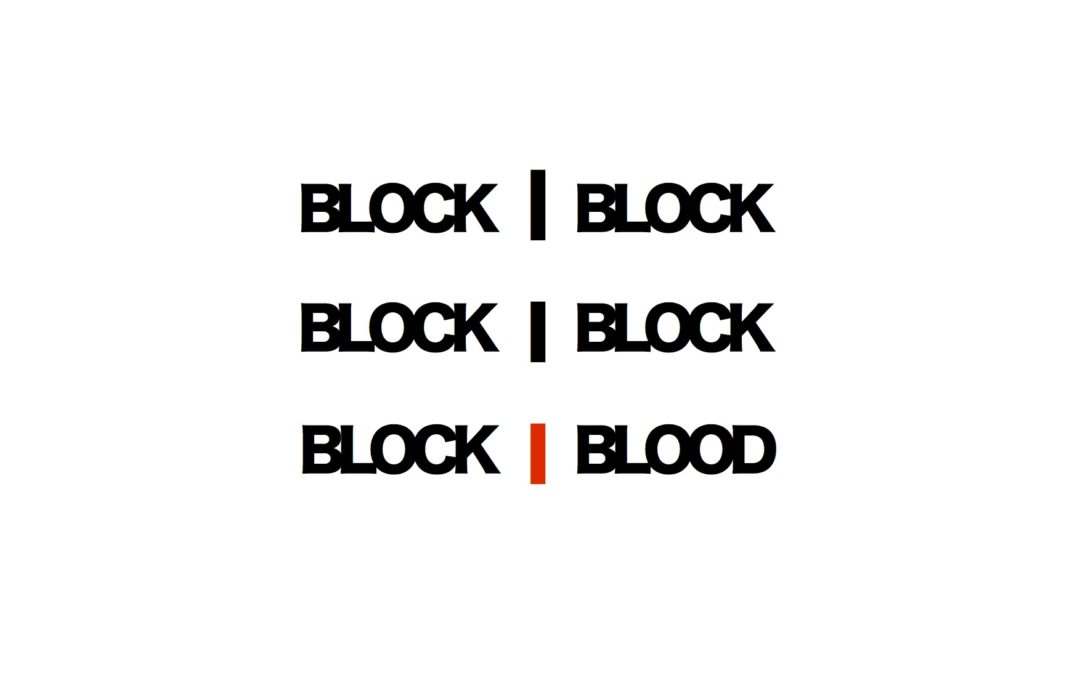The image is a graphic featuring three lines of all-caps black text on a clean white background, with the words appearing equidistantly. Each line comprises two words separated by a vertical line. The first and second lines each read "BLOCK | BLOCK" with a solid black vertical line in between. The third line reads "BLOCK" on the left side, separated by a red vertical line from the word "BLOOD" on the right side. This arrangement gives a distinctive appearance, with the major variation being the color change in the vertical divider and the substitution of "BLOCK" with "BLOOD" in the third line.